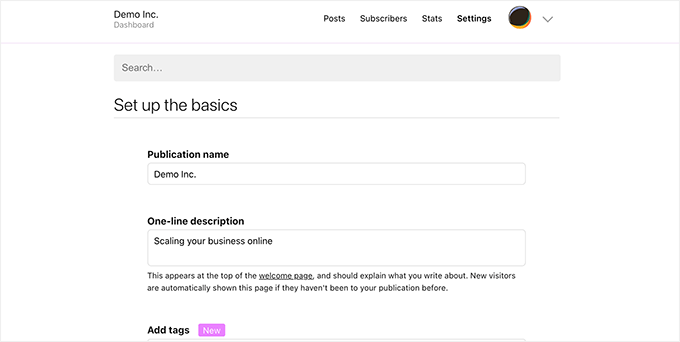The screenshot displays a template interface against a white background. At the top, a navigation bar prominently features "Demo Inc." on the left, indicating it might be a demo template. Adjacent to the site branding, the navigation menu includes tabs labeled "Dashboard," "Posts," "Subscribers," "Stats," and "Settings." To the far right of these tabs is a black circle followed by an inverted triangle, suggesting the presence of a drop-down menu.

Below the navigation bar, there is a gray search bar with the placeholder text "Search." Proceeding down the page, the first section is titled "Set Up the Basics." This section includes a field labeled "Publication Name," which is pre-filled with "Demo Inc." There is also a secondary field labeled "One Line Description" containing the text "Scaling Your Business Online."

An explanation follows this field, stating that this information appears at the top of the welcome page and advises the user to explain what the publication is about. New visitors to the site will see this page if they have not previously visited.

At the bottom of the screenshot, the section "Add Tags" is featured, accompanied by a lavender rectangle with the word "New" written in white font inside it. The overall layout and text suggest this is a demonstration of a content management system dashboard.